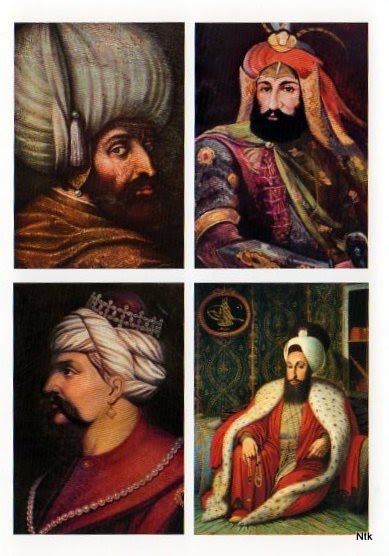This image features a composite of four vintage portrait-style photographs arranged in a window-pane format, with two images at the top and two at the bottom. Each quadrant contains a picture of a bearded man adorned in traditional and colorful attire, which may indicate some form of royalty or leadership. In the top left, the man wears a balloon-like hat and a formal dress coat, looking over his right shoulder. The top right displays a man in regal headgear with long, dangling ornaments and a vibrant jacket. The bottom left portrait shows a man in a dark maroon garb with a turban on his head. The bottom right image features the same man sitting on the floor with his hands outstretched, adorned with white hair, a crown, an earring, and red jackets in varying styles. The portraits are rich in colors including white, off-white, gray, brown, red, yellow, blue, purple, and maroon, and the overall presentation suggests a collection of significant historical figures. There is no text in the image to provide additional context.